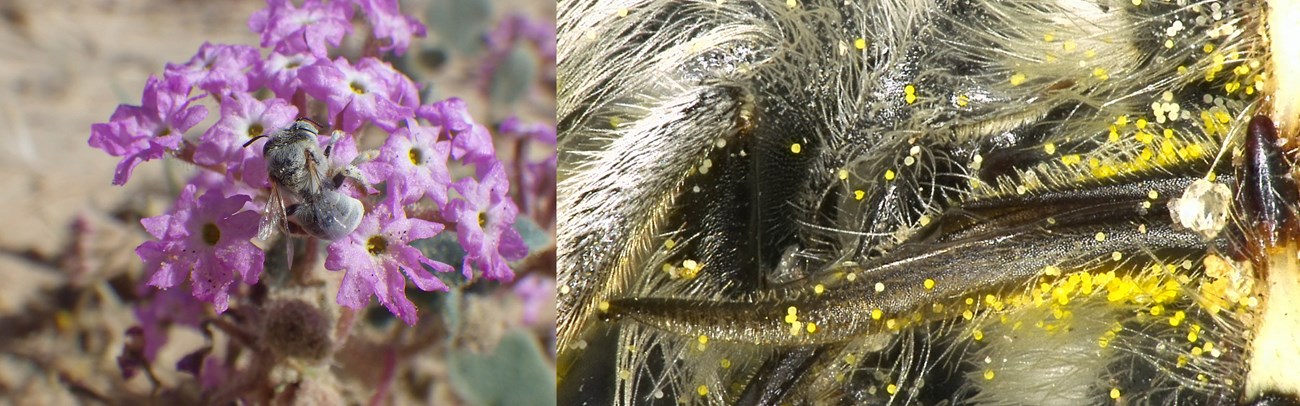This image is a rectangular two-panel photograph displaying two distinct scenes, both focused on bees in the context of pollination. 

On the left side, there is a bee (or possibly two bees) perched on top of a cluster of small, purple flowers with white centers. The scene is framed by a blurred, brownish, and somewhat desert-like background, suggesting the photograph was taken outdoors. The bee's back is visible, showing parts of its wings and antennae as it leans into the flower, participating in the pollination process. 

On the right side, a close-up photograph captures the intricate details of the bee's body. The image zooms in on the dark, blackish body of the bee, accentuated with reflective white hairs. Numerous yellow pollen grains cling to these hairs, resembling glowing dots. These pollen-covered fibers, along with strands that look like white feathery hairs, suggest a meticulous design, potentially created with software like Photoshop or through AI, evoking an almost artistic depiction of the pollination process. The background in this close-up is non-descriptive, focusing solely on the bee and its pollination role.

Together, the two images provide a detailed and striking visual exploration of bees engaging in pollination, from the broader view of bees on flowers to an extreme close-up of pollen-covered bee anatomy.